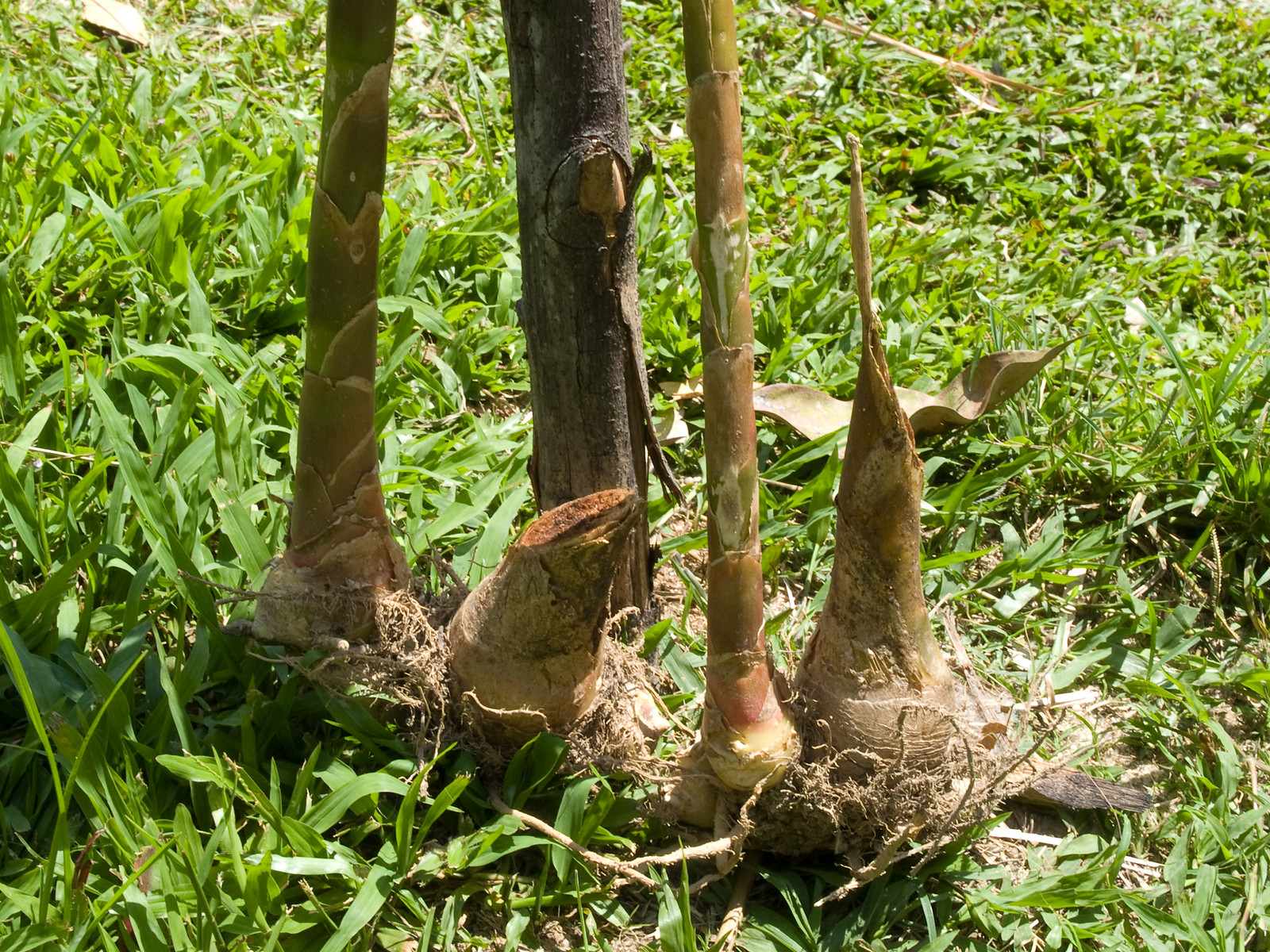This vibrant outdoor photograph, taken on a bright, sunny day, showcases a detailed close-up of the ground-level section of several tree trunks and vegetation. The background is lush with green grass, sporadically dotted with a few fallen, beige leaves. At the center of the image, four tree trunks stand prominently. On the left side, there are two dark brown tree trunks positioned closely together. In front of these, a sawed-off stump is visible, cut at an angle. Adjacent to these, to the right, is a thinner tree trunk with a beige hue and green markings. Further to the right, there is a stump of a broader trunk that appears to have been broken off, with only a small portion of the trunk remaining and a diagonal piece of wood sticking up from it. Interspersed among the tree trunks are various plants, including one with green and brown leaves and visible brown roots, along with remnants of brown stalks.